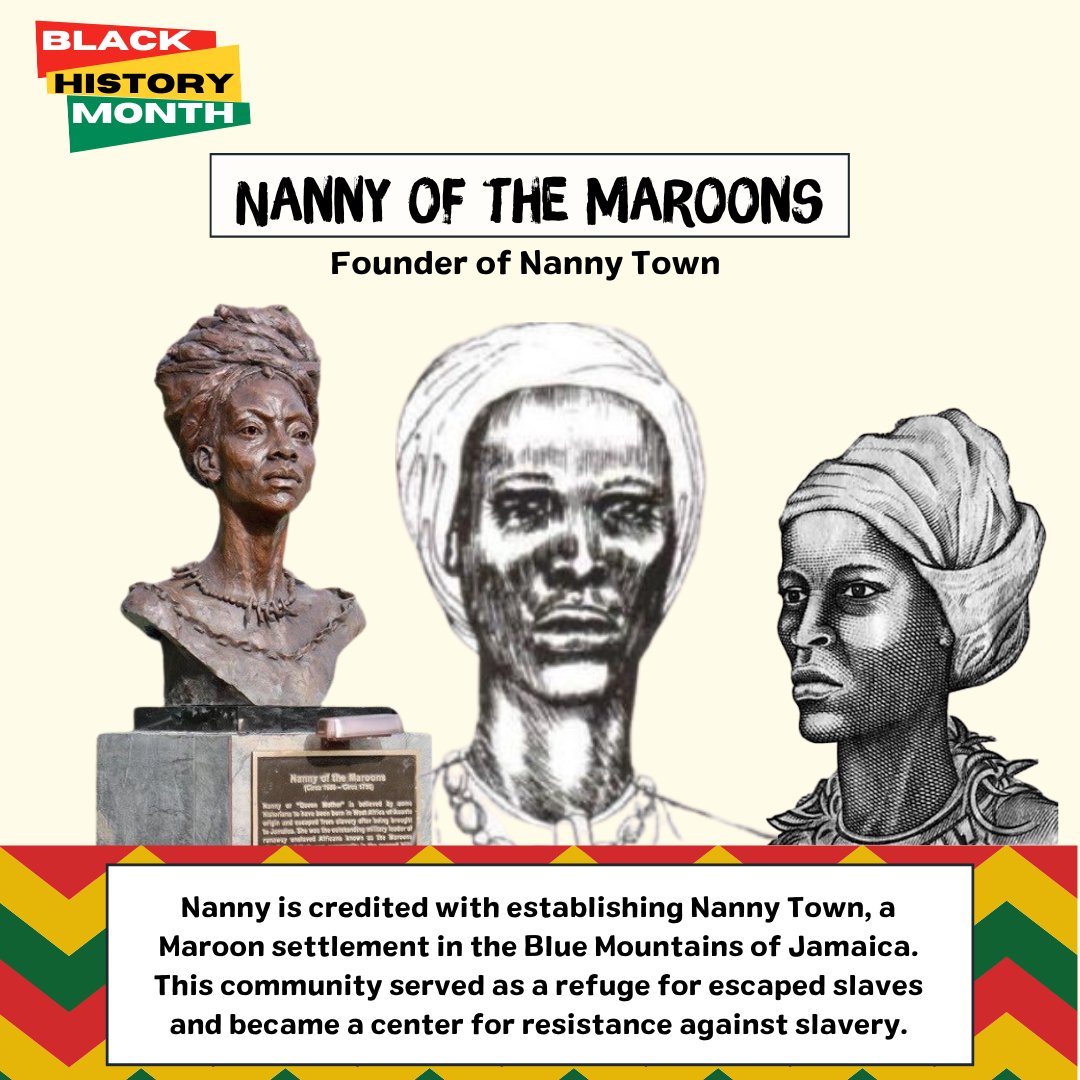The image is a poster commemorating Black History Month, highlighting Nanny of the Maroons, an essential figure in Black history. In the upper left corner, the words "Black History Month" are prominently displayed against a background featuring the colors red, yellow, and green. The centerpiece of the poster features the name "NANNY OF THE MAROONS" in bold, uppercase black letters within a white horizontal rectangle, with "Founder of Nanny Town" in smaller black type just below.

Below the title, the poster showcases three representations of Nanny of the Maroons. On the left is a statue depicting a bust of her head, neck, and shoulders, made of brown material and set on a concrete base. The middle image is a less defined pencil sketch of Nanny, where she is depicted wearing a white turban and attire. The rightmost depiction is a much more detailed pencil sketch, presenting her with a headdress and capturing finer facial features.

At the bottom, a large white horizontal rectangle, set against a vibrant chevron pattern of red, yellow, and green, provides key historical information about Nanny. The text explains that Nanny is credited with establishing Nanny Town in the Blue Mountains of Jamaica. This Maroon settlement served as a sanctuary for escaped slaves and became a hub of resistance against slavery. The background setting is bright and colorful, enhancing the clarity and visibility of the poster.